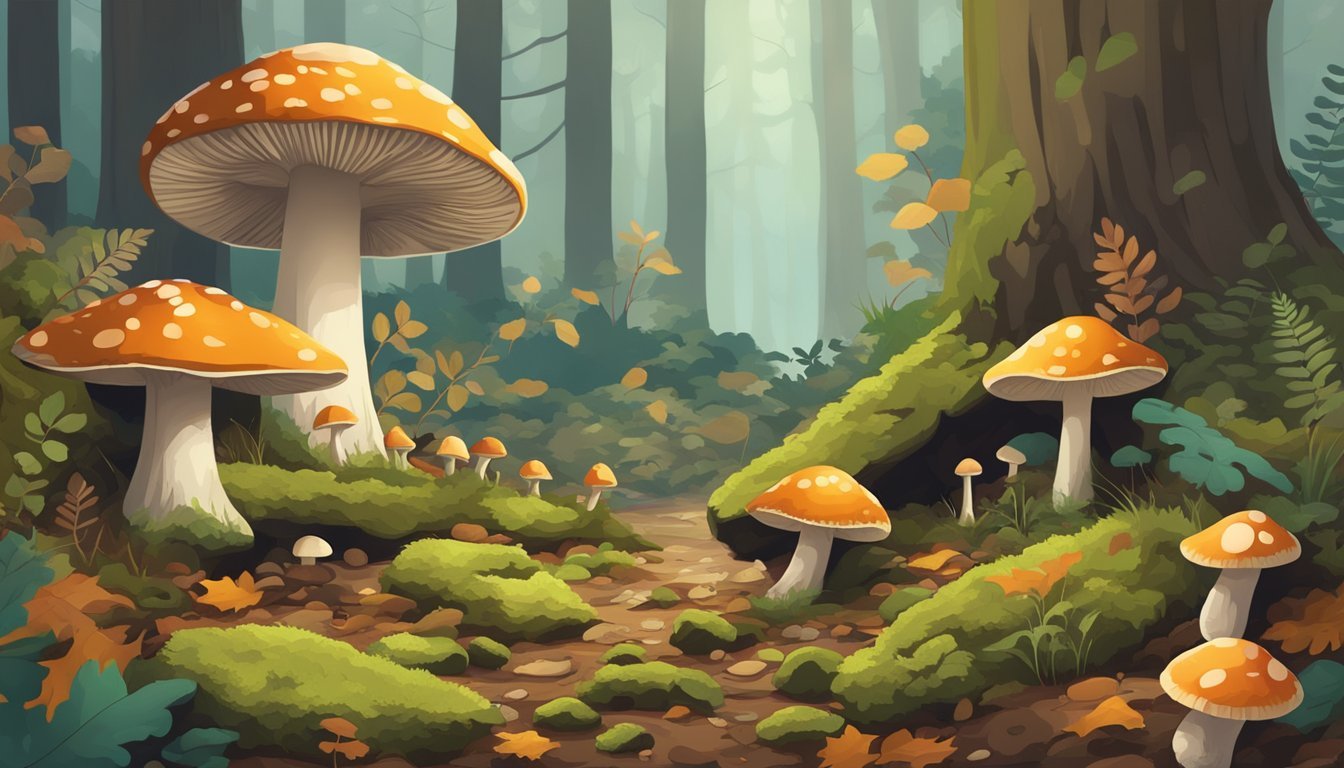In this digitally created, up-close, cartoonish painting of a forest scene, an array of vibrant orange and red mushrooms with white speckles on their caps dominates the focus. The mushrooms are arranged in the center foreground, with tall, bright white stalks supporting them. Among these, two notably large mushrooms stand prominently on the left, while several medium, small, and tiny mushrooms flank them, with the smaller ones nestled closely under the larger caps. The ground is a rich, textured mosaic of variously colored leaves—green, brown, white, and gray—interspersed with green vegetative brushes, sticks, and chunks of moss. The scene extends into the distance where tall tree roots and trunks, some with moss, reach vertically, culminating in towering, fog-enveloped pine trees. The atmosphere is misty, with a faint light piercing through the fog, adding a mystical aura to the forest. To the right of the composition, more mushrooms, smaller in size, and a significant tree trunk accentuated with moss contribute to the lush, detailed landscape that draws the viewer into the enchanted woods.